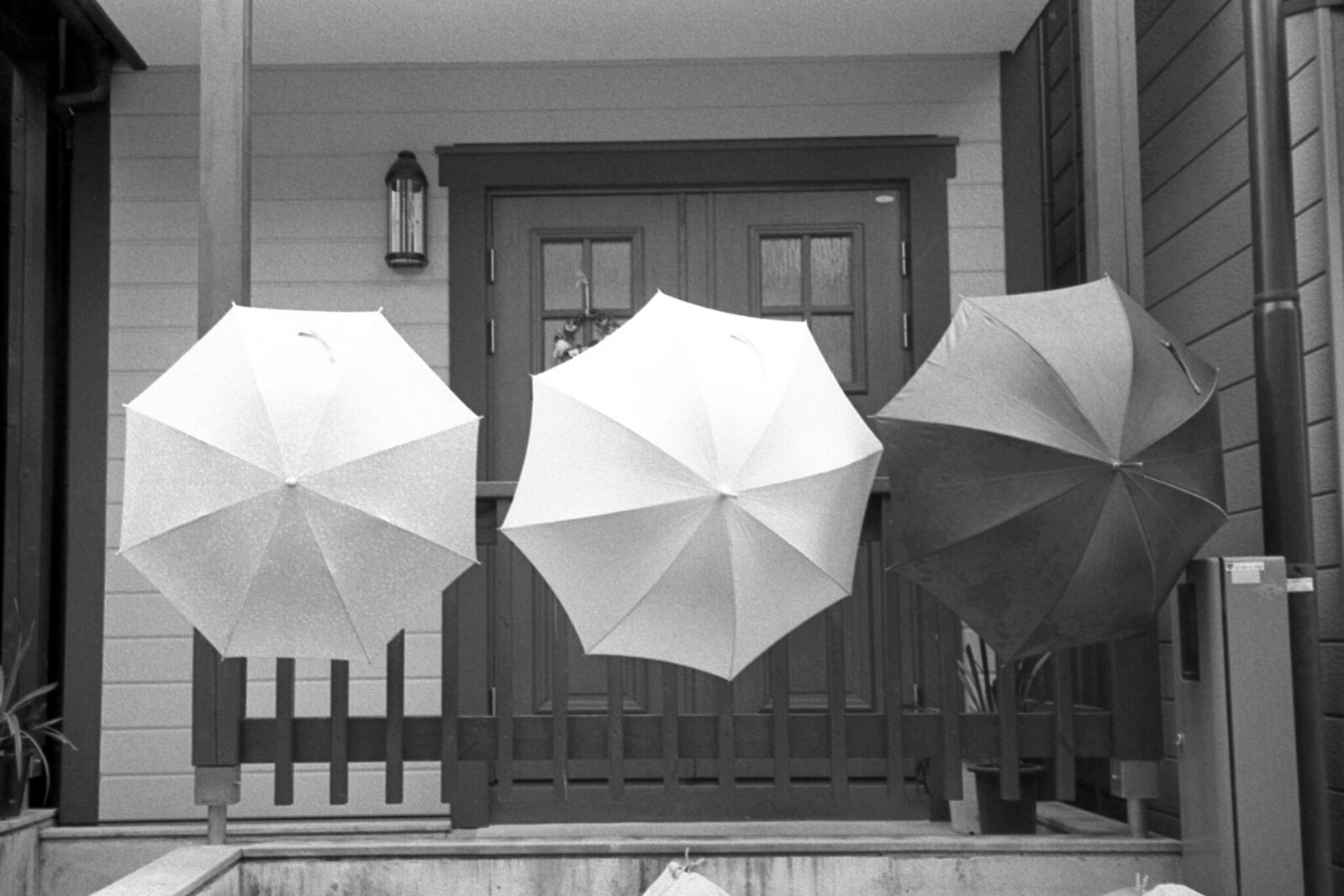The grayscale photograph displays a cozy entryway of a house, showcasing an intricate interplay of textures and elements. Centered in the image is a double wooden door with small windows at the top, creating a welcoming focal point. Flanking the doorway, a wooden railing of what appears to be a small porch or balcony prominently features three open umbrellas hung through its slats. The umbrellas, arranged from left to right, unfold in a sequence of light to dark shades: the first is likely pastel or light-colored, the middle one is white, and the rightmost umbrella is dark, perhaps black. Above and to the left of the doors, a light post or lantern adds a quaint touch. Below the umbrellas and the wooden railing, a stone wall is partially visible, with what seem to be the tops of sacks peeking over it. Further details reveal scattered house plants at the bottom left and right corners and hints of differing shades of grey on the wooden paling and siding that constitutes the house's facade. This careful composition and rich detail create a serene and homely atmosphere.